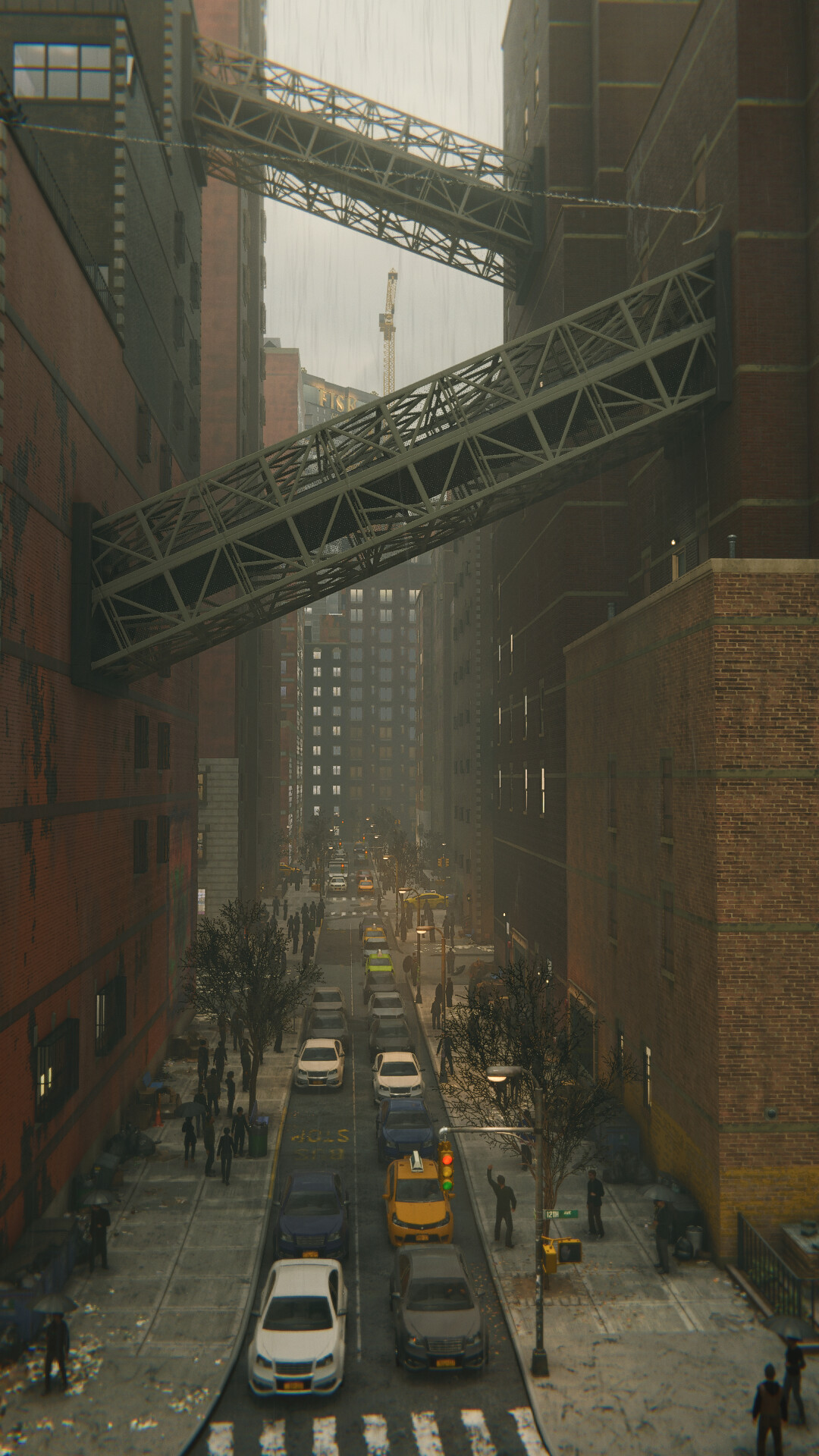In this highly detailed and realistic city scene, the photograph captures a densely populated urban block enveloped in a hazy, possibly polluted atmosphere. On both sides of the street, towering brick buildings dominate the landscape, interconnected by metal walkways. The first metal walkway extends from the red brick building on the left to a similarly imposing structure on the right, forming a pathway above the street. Further down the road, a taller section of the building on the right continues this theme with another elevated beam bridging back to the left building.

Numerous windows adorn the facades of these buildings, adding to the architectural complexity. Adding a touch of nature, trees line the sidewalks and sporadically dot the roadway. A myriad of cars are trapped in a traffic jam, stretching along the street in a seemingly endless row. The sidewalks are bustling with people, most of whom are walking purposefully. In the midst of this urban hustle, a man stands on the road with his arm outstretched, presumably trying to hail a taxi. The image captures the vibrant yet chaotic essence of city life with its blend of human activity, architectural elements, and environmental nuances.